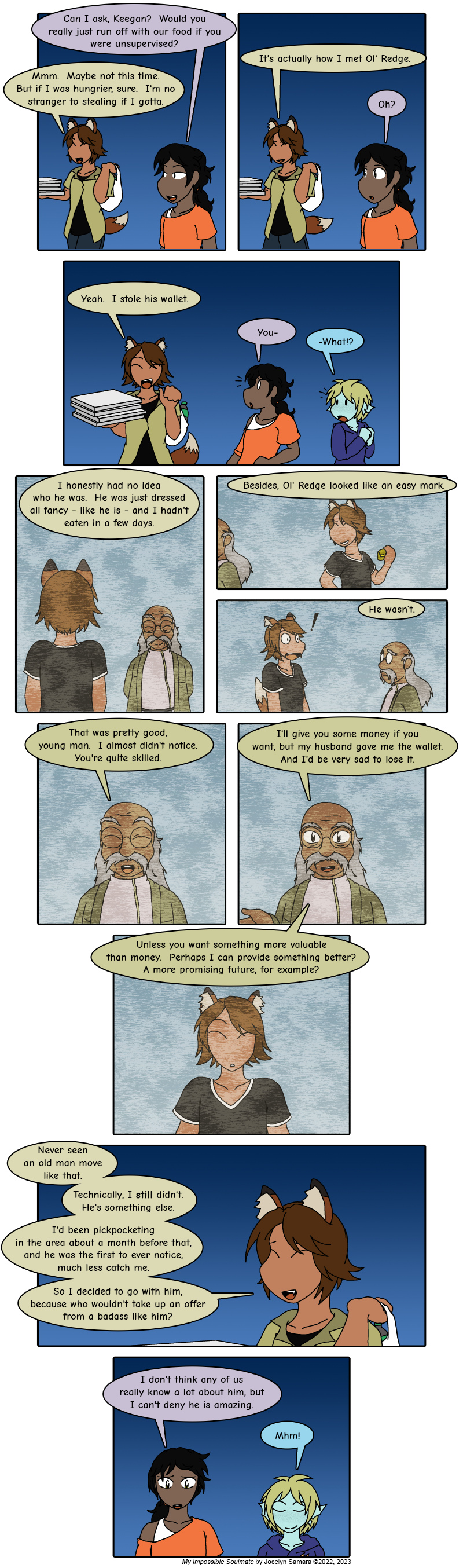The image is a vertically oriented comic strip composed of multiple panels featuring vibrant colors and detailed character illustrations. The strip showcases a recurring character, a woman with fox-like ears and tan skin, engaged in various dialogues. She appears alongside a diverse cast: a shorter woman with dark skin and dark hair tied in a ponytail, often seen in an orange shirt; a character with turquoise skin and blonde hair; and an elderly African-American man with gray hair. 

The background colors vary across the panels: the first three and the last two panels have a dark blue background, while the middle six panels have a mottled gray backdrop. Each panel contains word bubbles above the characters' heads, though the text is too small to make out. The top section introduces the main protagonist—the fox-like woman—interacting primarily with the dark-haired woman and the turquoise-skinned character. In the middle section, the focus shifts to an encounter between the fox-eared woman and the elderly man, spanning several panels. The comic strip concludes with the fox-eared protagonist again conversing with the dark-skinned woman and the turquoise-skinned character, mirroring the interactions from the beginning.